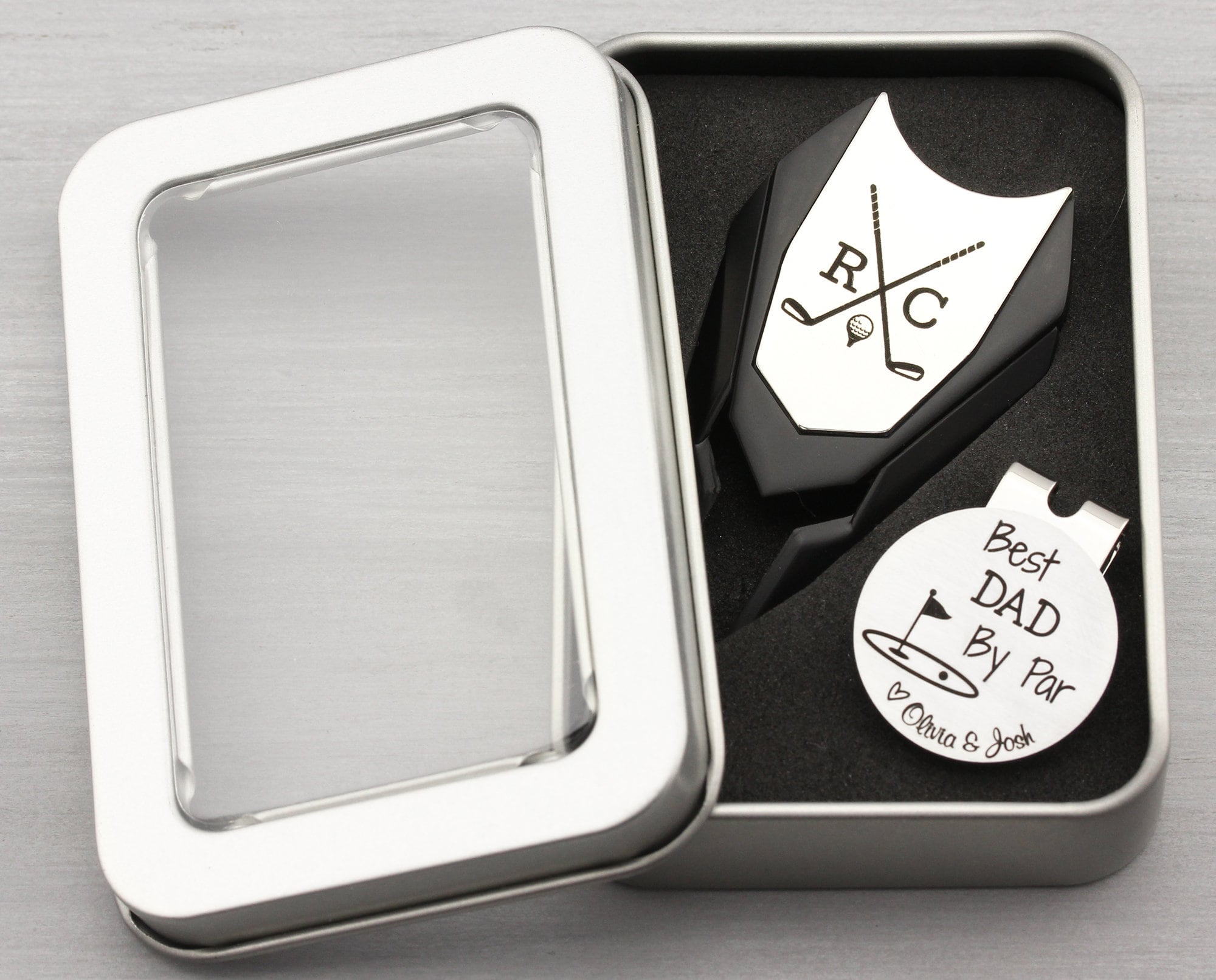The black and white image depicts a silver metallic gift box, rectangular in shape with rounded corners, lying on a wooden tabletop. The box has a clear plastic viewing window set into its lid, which lies separately to the left of the box. Inside the tin case, dark foam holds two items securely in place. The first item is a round metallic tie clip engraved with "Best Dad by Par, Hart, Olivia, and Josh," featuring an image of a golf green, complete with a flag and golf ball. The second item appears to be a golf-themed divot tool, possibly doubling as a key fob, with two crossed golf clubs and the initials "RC" engraved on either side of a golf ball sitting on a tee. This set, designed as a special golf-themed gift, emphasizes both functionality and a personal touch.